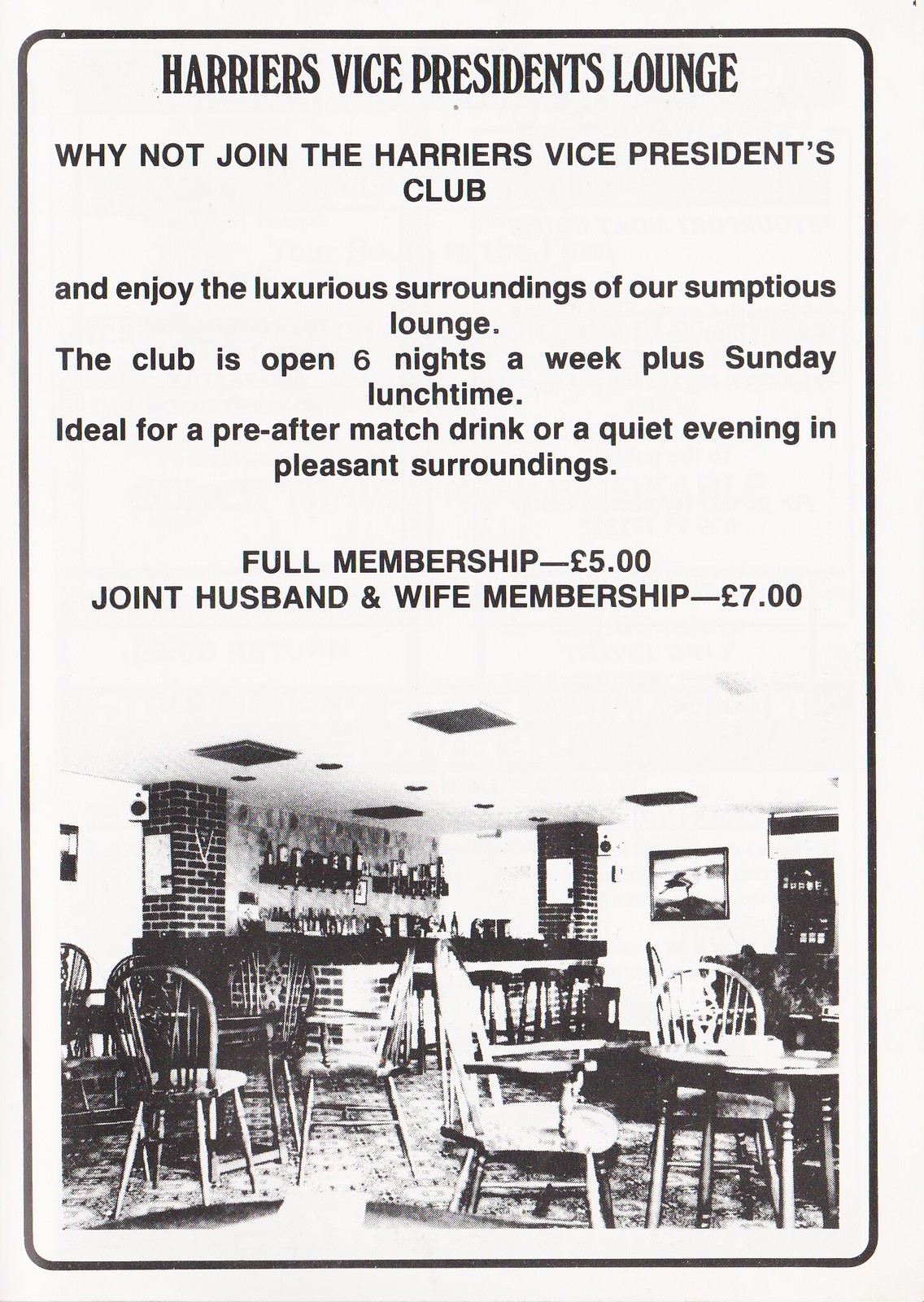The image is a vintage black and white advertisement for the Harrier's Vice President's Lounge. At the top of the poster, bold text reads, "Harrier's Vice President's Lounge" followed by a promotional tagline: "Why not join the Harrier's Vice President's Club?" Further down, the ad enticingly describes the lounge as a luxurious and sumptuous place, encouraging potential members to enjoy its opulent surroundings. The lounge is open six nights a week and Sunday lunchtimes, perfect for either a pre or post-match drink or for a quiet evening in pleasant settings. Membership details are provided, stating the full membership fee as £5.00 and a joint husband and wife membership at £7.00. The bottom of the advertisement features an image of the lounge’s interior, showcasing tables, chairs, a bar adorned with bottles of wine and other drinks, and brick details. Notably, black air vents can be seen on the ceiling. The overall style and monochromatic color scheme suggest the ad is several decades old, likely from 70 to 80 years ago, and adds a nostalgic touch to the promotion of this exclusive club in the UK.